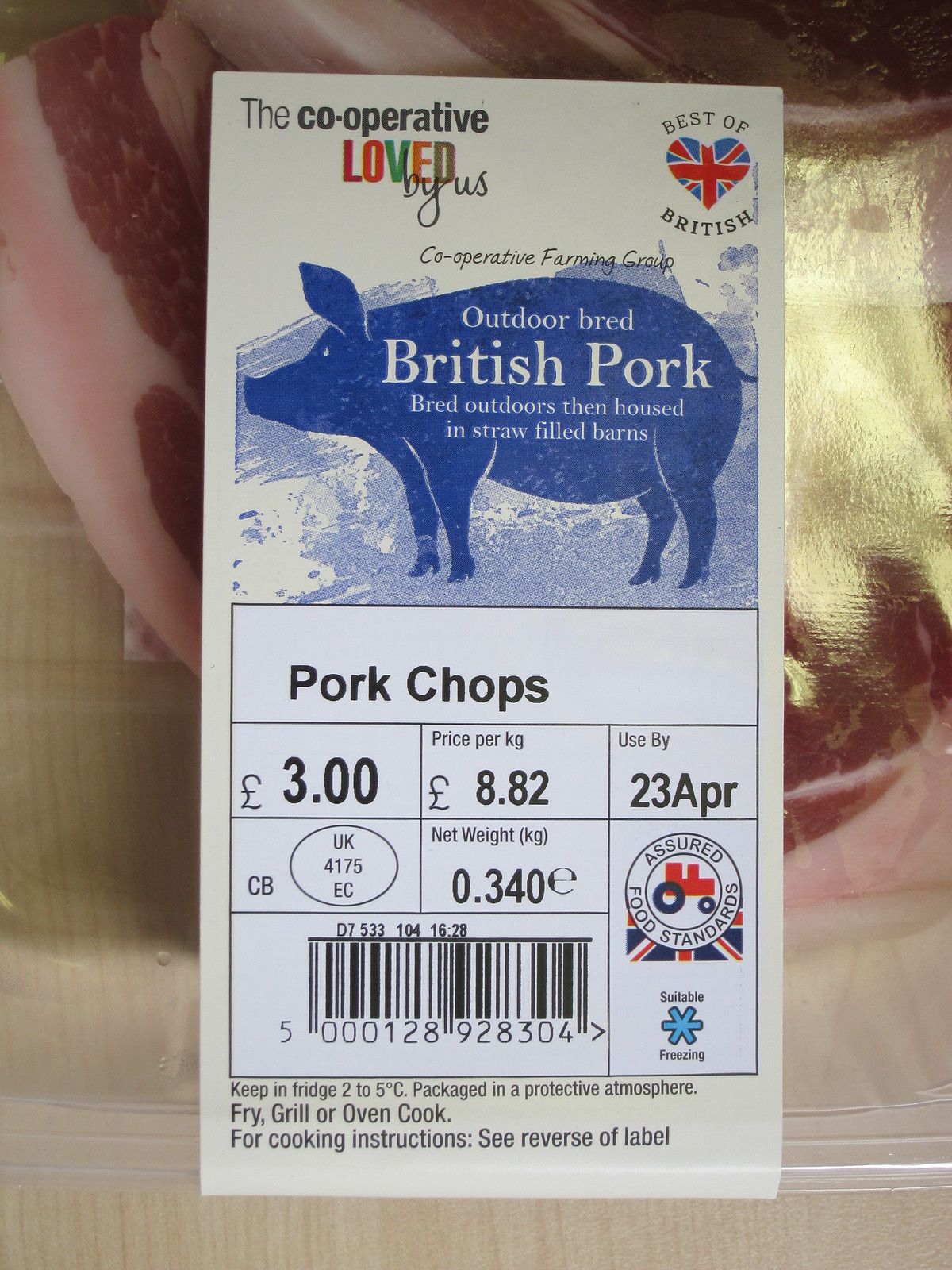The photograph is a detailed close-up of a packaged pork product, specifically pork chops. The meat is visible through a clear plastic container, showing its marbling and fat, and it rests on a light-colored wooden table or butcher block. The label on the package is predominantly white with numerous details. 

At the top of the label, in black text except for the multicolored word "loved," it reads "The Cooperative Loved by Us." To the right, the label features a heart-shaped Union Jack flag with the words "Best of British" underneath. Just below, it states "Cooperative Farming Group." 

Dominating the middle of the label, a blue pig is set against a light blue background, bearing the text "Outdoor bred British pork, bred outdoors then housed in straw-filled barns" in white lettering. Further down, a white box labeled "Pork Chops" provides additional information: the price is £3.00, the price per kilogram is £8.82, and the use-by date is 23rd April. The code UK 4175 EC is printed below the weight, which is 0.340 kilograms. 

On the right-hand side, a logo featuring a red tractor with blue wheels set against a British flag denotes the assured food standards. Next to this is a suitable-for-freezing symbol. At the bottom, black text on the khaki background advises to "Keep in fridge 2-5°C," and provides cooking instructions, encouraging consumers to fry, grill, or oven cook the pork chops. Additionally, instructions direct to see the reverse label for more details. On the left side of the label, a barcode is present.